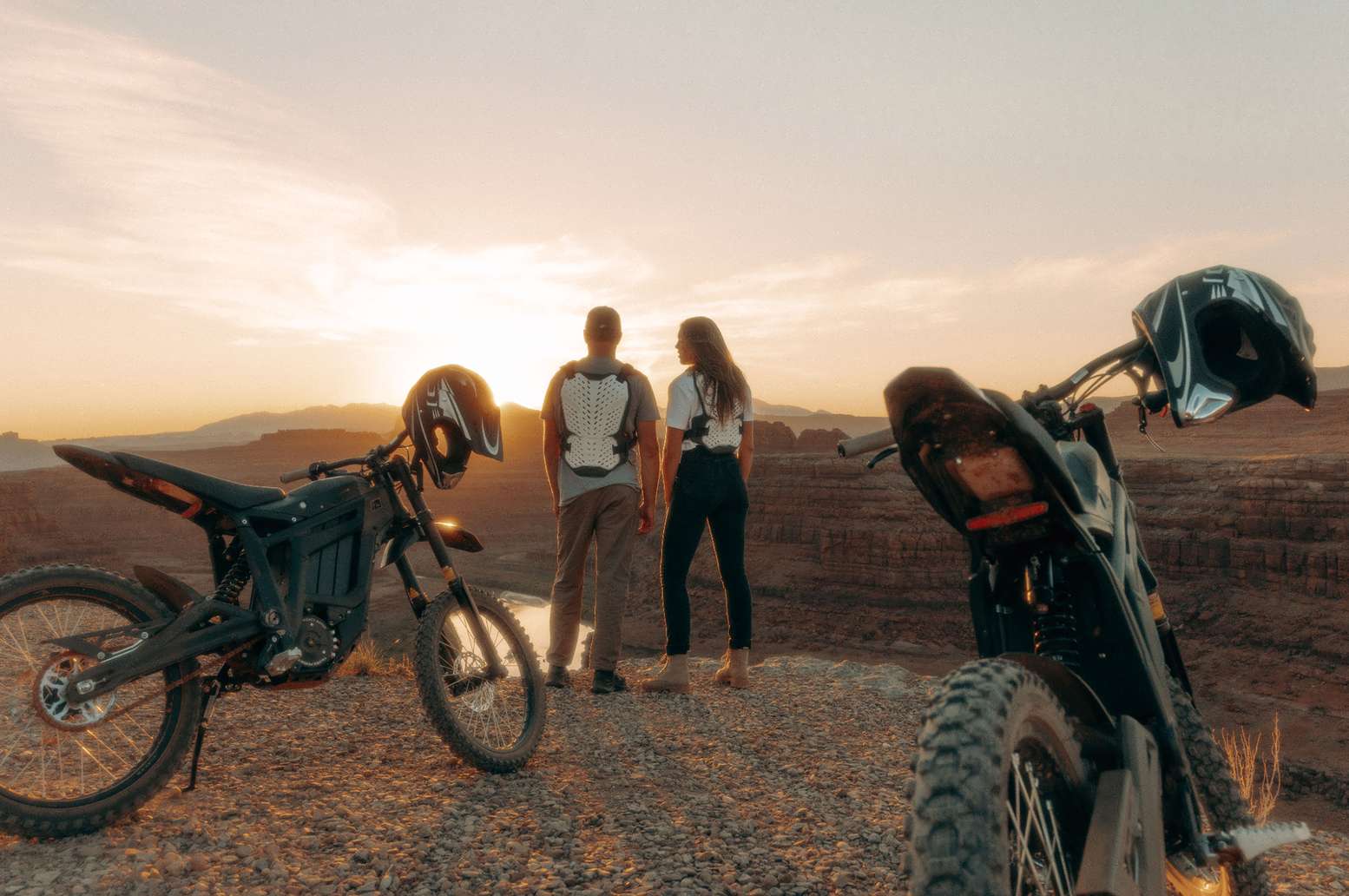In this captivating color photograph, a young man and woman stand side by side atop a cliff, overlooking a breathtaking scene that closely resembles the Grand Canyon at sunset. The sky is painted in hues of light orange and pink, with the sun a brilliant white-yellow spot just above the horizon. Both individuals are equipped with motorcycle-type protective vests; the man is dressed in tan pants and a gray t-shirt, while the woman wears a white t-shirt, black pants, and tan boots. Each has a helmet resting on the handlebars of their black electric motocross bikes, identifiable by their lack of traditional gas-powered engines and distinctive red stripes on the rear fenders. The majestic view captures the deep, cavernous expanse of the valley below, with a river reflecting the diminishing sunlight as it winds through the canyon.